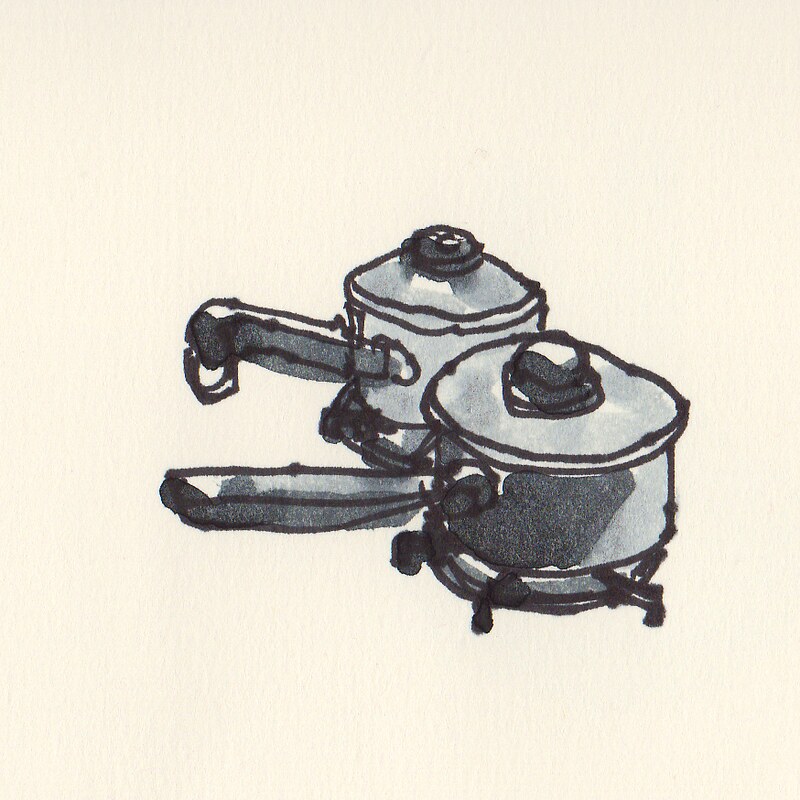This image features an intricately detailed, watercolor-esque painting or drawing of two stovetop pressure cookers set against an off-white background. Both pots are depicted in shades of light and dark gray, with black ink outlining their forms. The pots are arranged in a stacked formation, one slightly behind the other, each sitting on what appears to be black gas stove burners or trivets. The top pot has a black knob on its lid and a long, black handle that extends to the left, featuring a ring hanging off its end. The pot beneath it also has a black knob on its lid and a long, dark grey handle. Both handles and lids exhibit a blend of watercolor and marker strokes, adding depth and texture to the image. The rounded, cylindrical shapes of the pots contrast with the angular lines of the burners, which consist of circular frames supported by legs extending outwards.